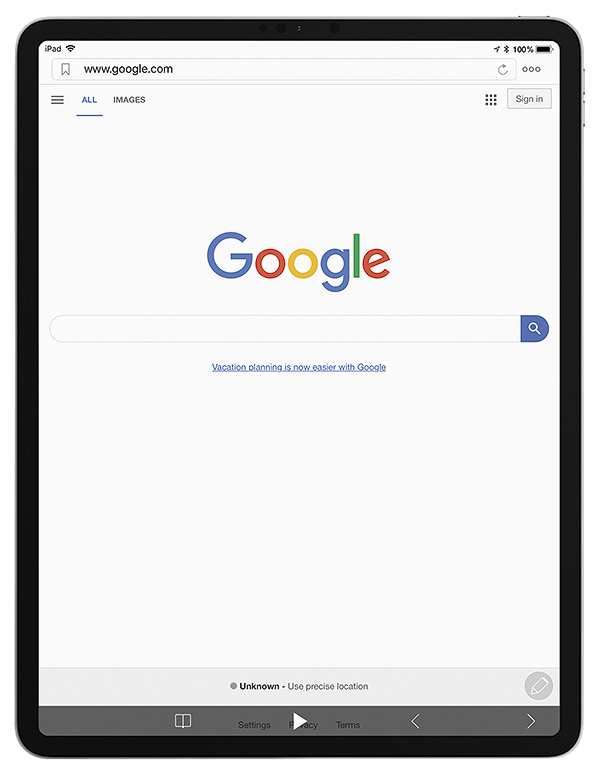This image is a detailed screenshot of an actual iPad. The device features the characteristic thin black bezel and rounded aluminum or stainless steel edges. The interface prominently displays the iPad's on-screen elements. 

In the upper left corner, the status bar shows "iPad" alongside the Wi-Fi icon. On the upper right, there are icons indicating location services (an arrow), Bluetooth status, and a full 100% battery life. 

Just below the status bar is the URL bar of the Safari browser, showing the address "google.com." The URL bar includes three dots for additional options and a reload button. 

Dominating the center of the screen is the Google homepage. The well-known "Google" logo, displayed in blue, red, yellow, and green, is positioned above the central search bar. Beneath the search bar, there is a blue hyperlink stating, "Vacation planning is now easier with Google." 

At the very bottom of the screen is a gray footer containing text that reads, "Unknown precise location," along with links to "Settings," "Privacy," and "Terms." 

Additional User Interface (UI) elements are present, suggesting that the screenshot might have been taken from a prototyping or development environment.